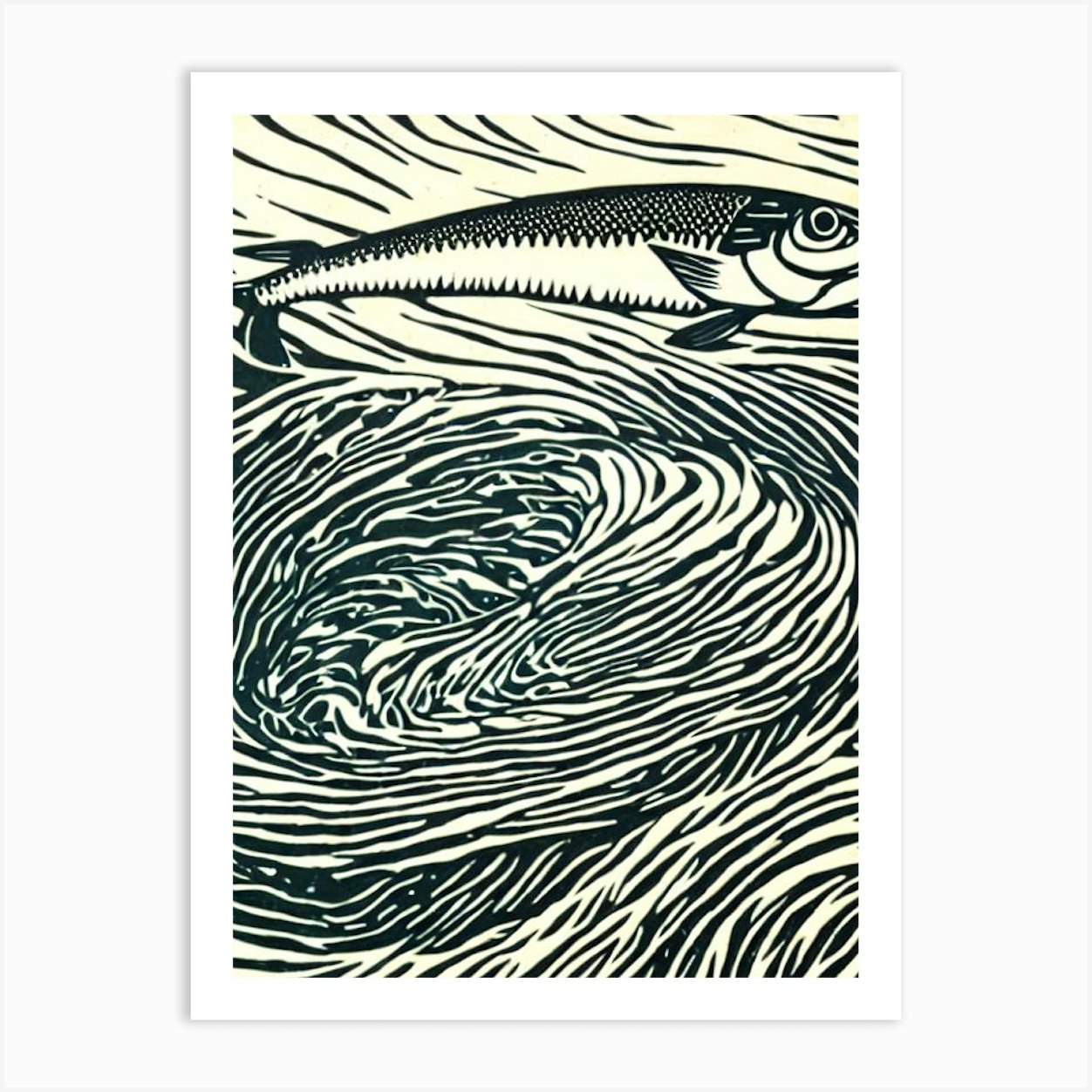This is a meticulously detailed drawing, artistically framed in white with subtle shadowing along the edges for a three-dimensional effect. At the center, a beige square background creates a stark contrast, accentuating the flowing black lines that mimic the appearance of running water. The composition features thicker, more pronounced lines cascading from top to bottom, with wider, more expansive spaces concentrated at the top.

In the upper section of the image, a fish is meticulously drawn with its mouth partially cut off by the frame, creating a dynamic and engaging focal point. The fish's head is broad, tapering elegantly towards the tail, which is also slightly cropped on the left side of the picture. The artist has captured intricate details, including delicate lines on the fins and a fin positioned underneath the head. The fish's eye, marked in black, adds depth and realism. The overall attention to detail in this artwork brings the aquatic subject to life, emphasizing its natural beauty.